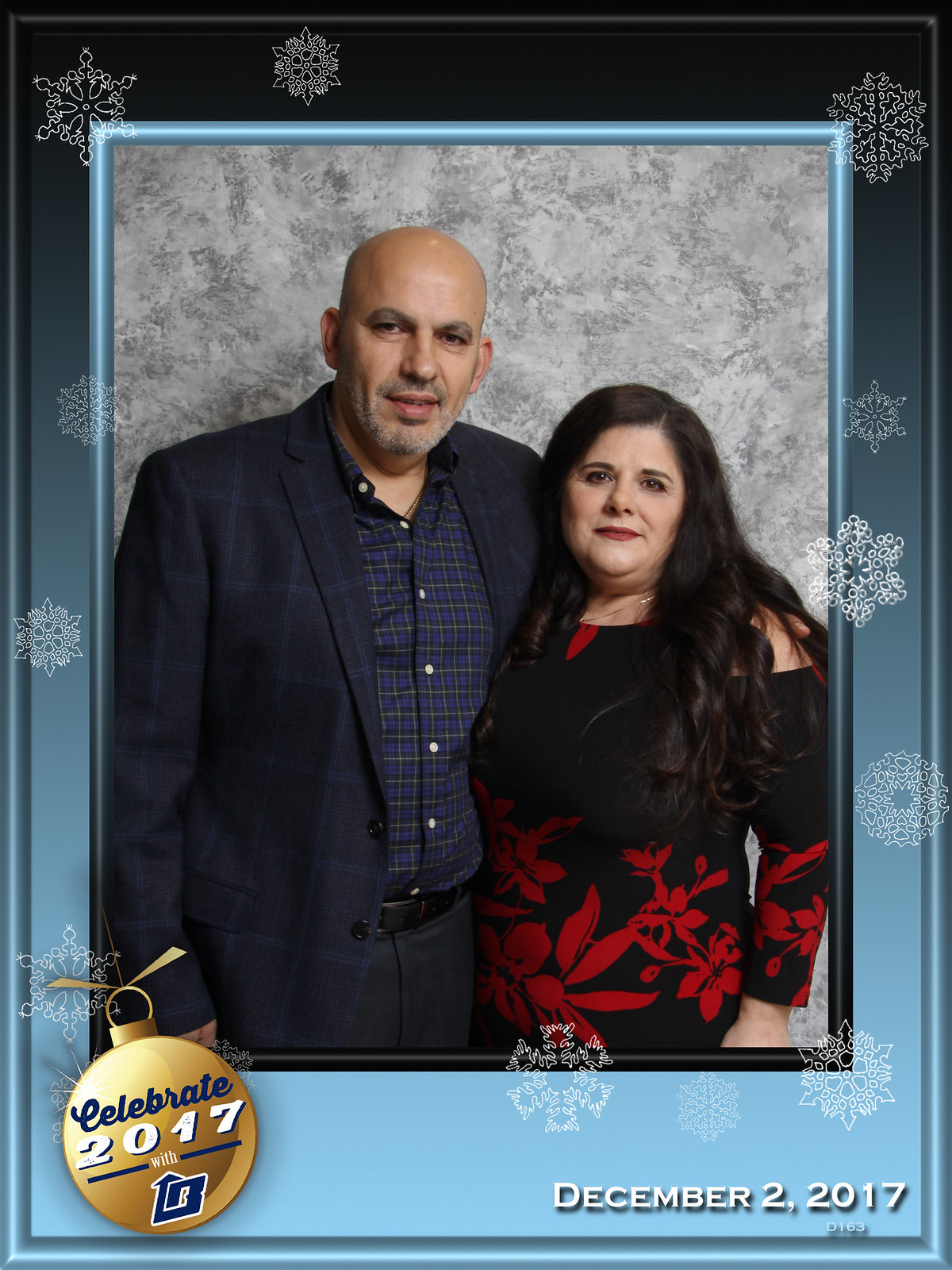This is a professional portrait of a couple, likely in their 40s, set within a festive graphic frame. The man, who is bald with a graying goatee, is on the left and has a light complexion. He wears a navy blue plaid suit over a similarly patterned checkered shirt with shades of green and blue. His left arm is around the woman beside him. The woman, slightly shorter than the man, has long, dark brown hair that extends past her shoulders and wears lipstick. She is dressed in a black long-sleeved top adorned with red floral patterns. Both appear neutral as they face the camera. The background is mottled gray, surrounded by a dark-to-light blue frame adorned with white snowflakes and a gold Christmas ornament graphic. In the bottom right corner, the text reads "December 2nd, 2017," while the bottom left features the wording "celebrate 2017 with" alongside an indeterminable logo. The overlay makes the frame seem like part of a digital holiday card, possibly intended for email distribution.